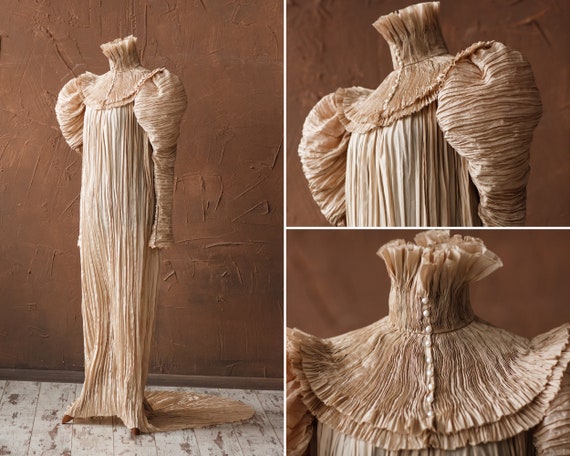The image is a collage showcasing a single Victorian-style dress from the 1800s, displayed on a mannequin without a head. The centerpiece of the collage is a full-length photo of the dress, which reveals its intricate design and extends from below the bust to the floor, with a train that drags on the ground behind it. The dress features vertical brown and white pleats, with puffy shoulders that taper down the arms. The frilled neckline, adorned with ruffles that rise up the neck, adds to its historical elegance, further accentuated by pearl buttons running down the center top of the dress. The right side of the collage consists of two close-up images: the top close-up focuses on the crumpled, puffy shoulders, and the bottom close-up highlights the frilly neckline and the shoulder details. The background includes a brown wall and a white and gray floor.